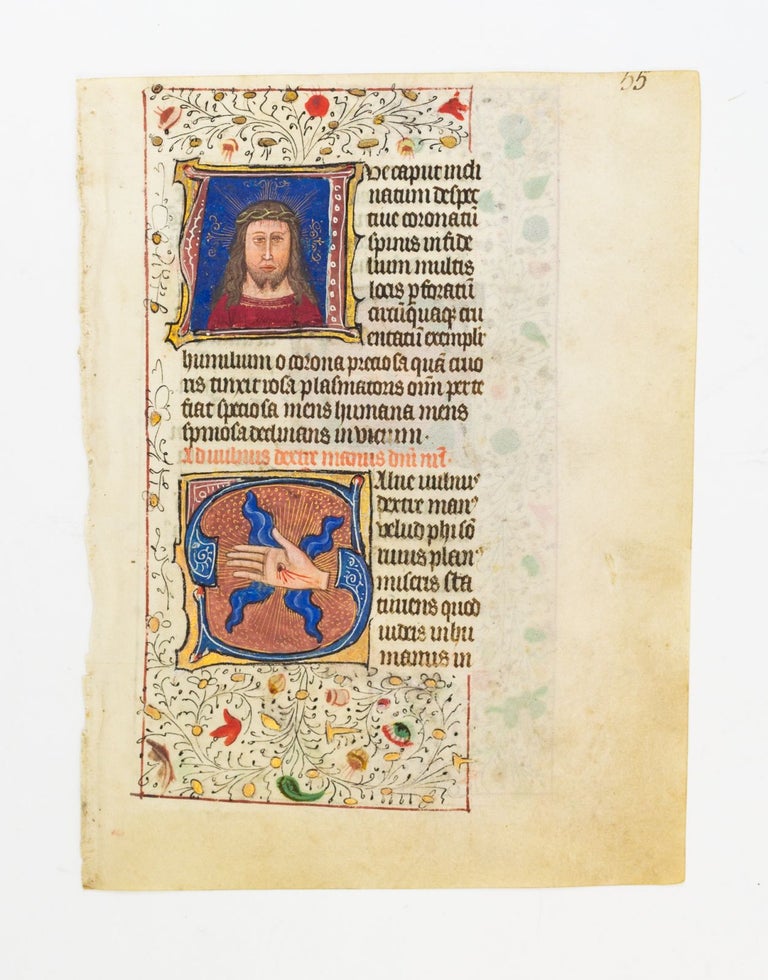The image depicts an old, worn, and yellowed page, likely torn from a medieval manuscript or book, with a rustic, beige appearance indicative of its age. The page is in a vertical orientation featuring a gray background, with a distinct tear on the left-hand side. The top right corner is marked with the number "55." The layout includes intricate floral patterns with long-stemmed red, orange, and yellow flowers framing the text throughout the page and a red border encompassing most of the content except on the right side where some text extends beyond the border.

The page contains two color illustrations central to its composition, depicting Christian themes. The first is an image of Jesus Christ, portrayed with long hair and wearing a red robe and a crown of thorns, facing the viewer head-on. Below this, a second illustration depicts a hand with a visible wound, bleeding, symbolizing the Crucifixion. The textual content, wrapping around these images, appears to be in a foreign, likely Latin, language. Red text appears mid-page, adding emphasis to certain words. The detailed floral and textual arrangement suggests this page narrates events from the life of Jesus, specifically his crucifixion, making it a significant Christian artifact.